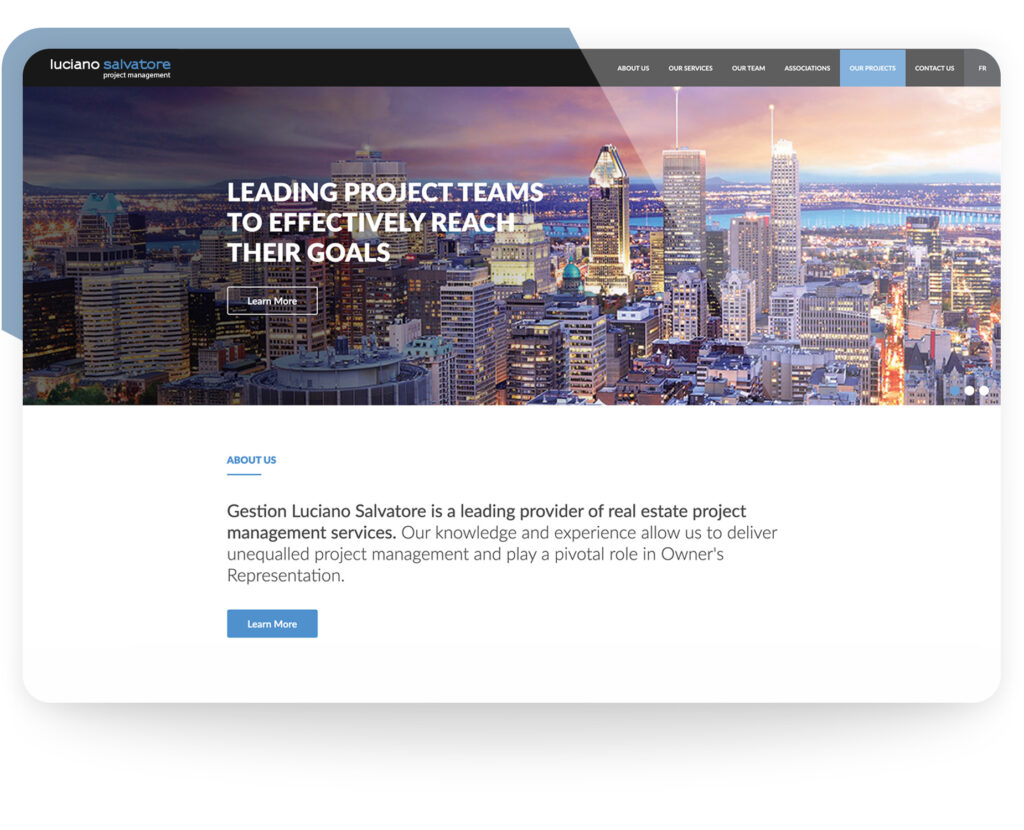The image features a detailed and dynamic layout, divided primarily between a left-hand blue-gray section and a right-hand black section. The blue-gray portion begins slightly to the right of the midpoint at the upper edge, curving around the upper-left corner, and extending down to just above the midpoint on the left edge.

At the top of the image, spanning right to left, there is a black section with the name "Luciano Salvatore" prominently displayed. "Luciano" is written in lowercase white font, while "Salvatore" is in blue font, with smaller white text beneath it that's too small to discern.

Across the top of the image, white capitalized text lists several headings: "ABOUT US," "OUR SERVICES," "OUR TEAM," and a partially readable "ASSOCIATIONS." Following a diagonal transition from blue to a hazy right-hand area, the headings continue with "OUR PROJECTS" in turquoise and "CONTACT US."

Central to the image is a horizontal visual that spans right to left. On the left side, bolded white uppercase text reads, "LEADING PROJECT TEAMS TO EFFECTIVELY REACH THEIR GOALS." Below this text, a white-outlined box with "LEARN MORE" in the center is prominent. The left portion of this image is darker, transitioning to a brighter, slightly hazy right side. The background showcases a cityscape with tall, closely packed buildings, illuminated lights, and a dark sky on the left transitioning to a yellowish sky on the right. Water is visible in the background on the left side.

Towards the bottom left, in turquoise, the text "ABOUT US" is underlined with a turquoise line. Beneath it, in bold black font, reads "GESTION," followed by "Luciano Salvatore is a leading provider of real estate project management services." Non-bolded text below mentions, "Our knowledge and experience allows us to deliver unequaled project management and play a pivotal role in Owner's Representation," with "Owner's Representation" capitalized. At the bottom, another "LEARN MORE" box is visible, featuring white text against a blue background.